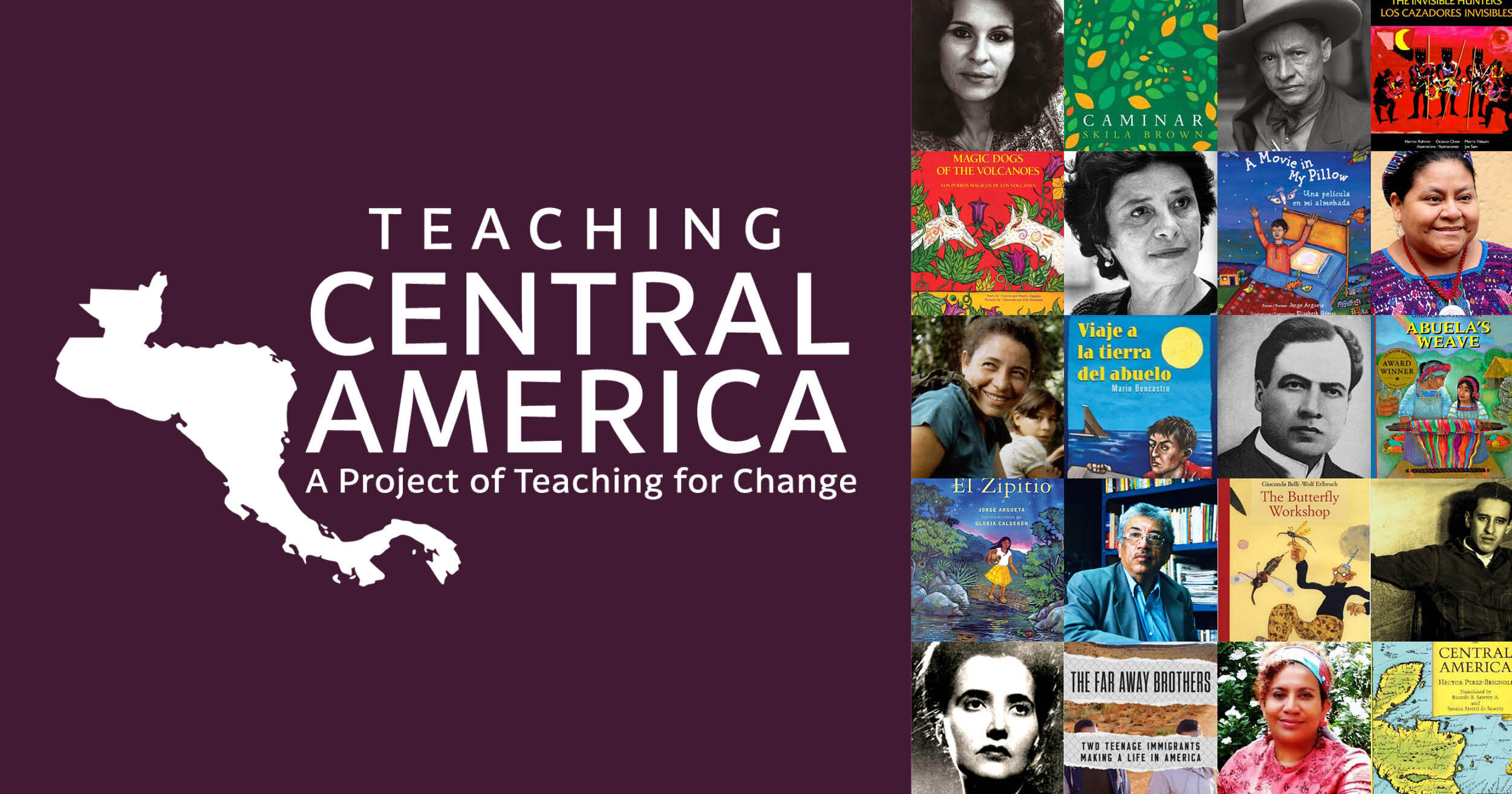This detailed panoramic image likely serves as an advertisement or poster. The left two-thirds of the image features a dark plum-colored background with bold, block white text stating "Teaching Central America, a project of Teaching for Change." To the left of this text is a white, silhouetted geographical representation of Central America. Moving to the right third of the image, there is a vivid collage composed of 20 elements arranged in a grid of five columns by four rows. This collage includes a mix of headshots, likely of authors or teachers, and colorful book covers, seemingly children's books. Among these, several black and white images are interspersed. Additionally, a small map appears in the lower right-hand corner of the collage, adding another layer of visual information to this educational and promotional piece.